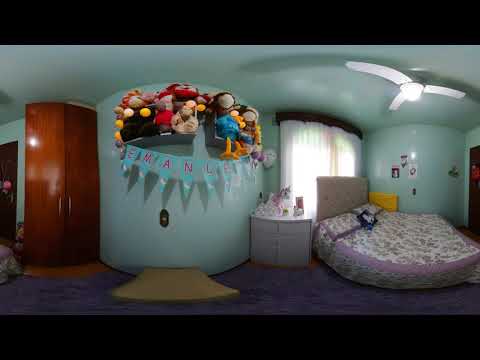The image depicts a uniquely shaped bedroom, characterized by its light turquoise (possibly due to lighting) walls and ceiling, with domed sections on the left and right. The room is anchored by a purple carpet and a ceiling adorned with a white, three-blade ceiling fan. Centrally, a purple floral-patterned mattress lies on the floor in front of a window dressed in a sheer white curtain. Next to the mattress is a small gray nightstand, holding various items including a toy unicorn. Above this nightstand, the domed wall showcases shelves brimming with stuffed animals, beneath which dangles a blue, triangular-sectioned banner. This banner partially spells out letters that seem to form "E-M-A-N-L-E." The room also features a tall, dark brown wooden wardrobe on the left side. Surrounding the space are additional personal touches like posters, a wallcloth, and an assortment of pillows—two matching the mattress and one blue—against an off-white headboard. This attention to detail, along with the presence of a double door and rich decor, suggests it might be a young person's vibrant, organized sanctuary.